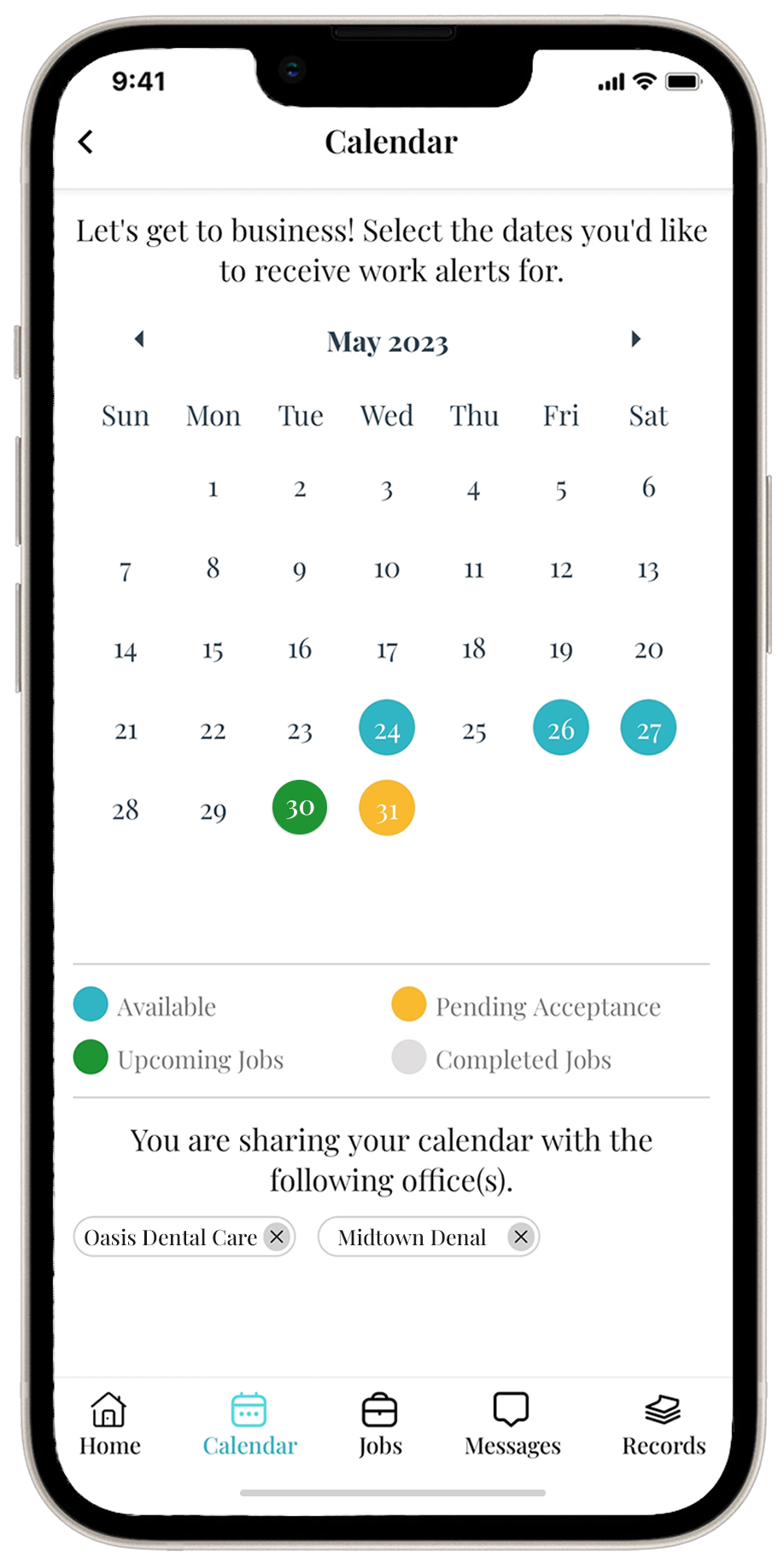The image depicts a cell phone displaying a scheduling app interface, presumably for temporary dental office work. The phone screen shows the status bar indicating the time as 9:41 AM, with full cell signal bars, Wi-Fi connectivity, and a fully charged battery. The app screen showcases a calendar view for May 2023 with various dates highlighted. Specifically, the 24th, 26th, and 27th are marked with blue circles, the 30th with a green circle, and the 31st with a yellow circle.

Below the calendar, a key explains the color coding: turquoise indicates availability, orange signifies pending acceptance, gray denotes completed jobs, and blue circles represent selected dates for receiving work alerts. An instructional line prompts the user to select the dates for work alerts, under the heading "Let's get to business."

Further down, options are available for sharing the calendar with specific offices, namely Oasis Dental Care and Midtown Dental Care, hinting at the app’s functionality for managing temporary dental work assignments. At the bottom of the screen, there is a navigation bar with icons for Home, Calendar, Jobs, Messages, and Records, with the Calendar icon highlighted in blue while the rest remain dark.

The entire phone, including its edges and buttons, is visible against a white background, suggesting this image might be a promotional material to demonstrate the app's user interface on their website.